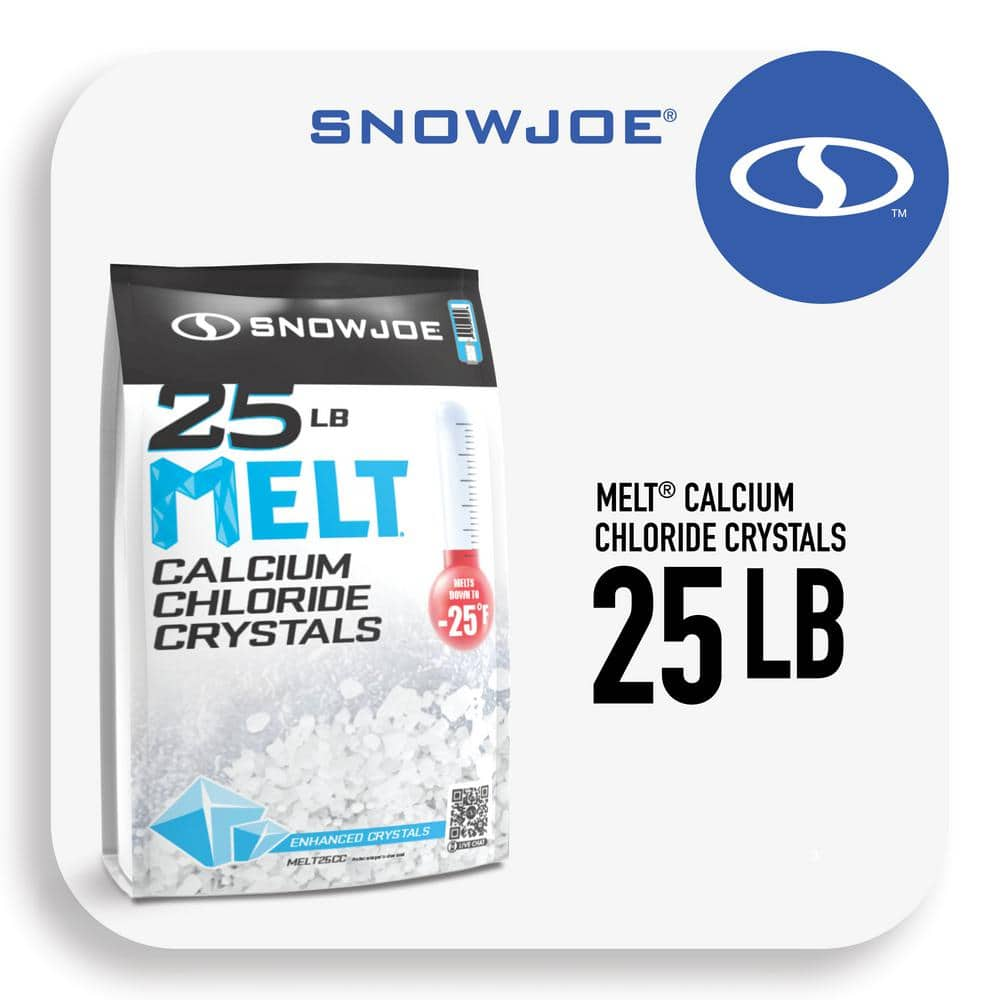The image is an advertisement on a white square background with rounded corners and a subtle shadow on the left side, giving it a 3D effect. At the top of the advertisement, "Snow Joe" is written in large blue capital letters, with a small registered trademark symbol above the 'E'. To the right of this text, there's a blue circle featuring a white oval and a white squiggly 'S' inside, which serves as the Snow Joe logo. 

On the bottom left of the image is a bag with a black top and white lettering reading "Snow Joe." Below this, "25 LB MELT" is prominently displayed in large blue letters, followed by "CALCIUM CHLORIDE CRYSTALS" in black letters. The term "MELT" is also highlighted on the bag in capital blue letters. Near the bottom of the bag is additional small text in black letters indicating "ENHANCED CRYSTALS."

To the right of the bag, a white thermometer with a red bulb at the bottom shows a reading of minus 25 degrees Fahrenheit (written as "-25°F"). Scattered at the base of the bag are white and blue-enhanced salt crystals. A QR code is also visible near the bottom right corner of the bag. 

Overall, the advertisement effectively communicates the product details of Snow Joe's 25-pound bag of calcium chloride melt crystals, emphasizing the brand's name, the product type, and its temperature efficacy.